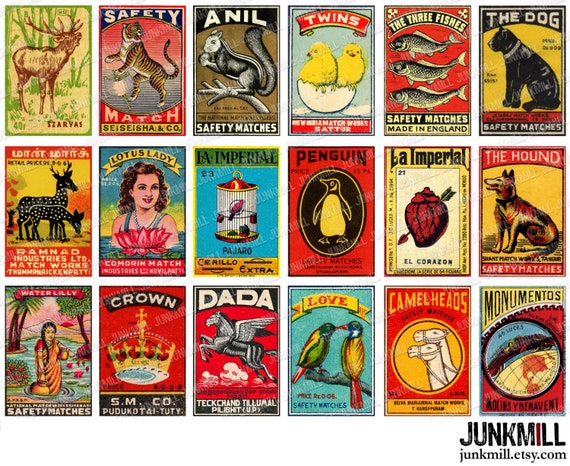This vibrant and colorful image showcases a collection of 18 vintage matchbox covers, meticulously arranged in three rows of six. Primarily hailing from India, as suggested by the language on some boxes and names of Indian companies like Ramnath Industries Limited, the collection also includes a few matchboxes marked "Made in England," reflecting a blend of origins. The covers feature a myriad of designs, many of which are hand-drawn and adorned with illustrations of animals and various motifs. Notable names include "Safety Match," "Sesisha & Co," "Anil," "Twins" with yellow birds, "The Three Fishes," "The Dog," "Water Lily," "Crown," "Dada," "Love," "Camel Heads," "Monumentos," and "Lotus Lady." The depiction maintains vibrant colors such as yellow, blue, black, red, green, white, and orange, enhancing the vintage aesthetic. A small watermark in the lower right corner reads "Junk Mill" and "junkmill.etsy.com," indicating the image advertising vintage poster prints available for purchase from this Etsy store.